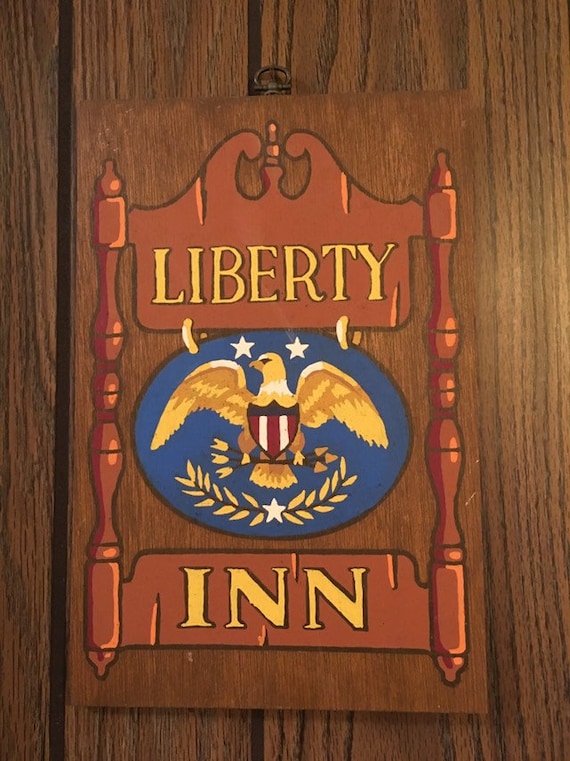The image is a colored photograph depicting a door with a glossy brown, lacquered wooden finish. Upon closer inspection, there appears to be a plaque affixed to this wooden surface. The plaque, rectangular and in a reddish-brown hue, stands out prominently. The plaque features a metallic hook at the top for hanging. On either side of the plaque, there are two vertical bars. The top part of the plaque prominently displays the word "LIBERTY" in bold, yellow capital letters, while the bottom part similarly reads "IN." Between these two inscriptions is a blue oval background containing an intricate emblem. This emblem showcases a golden eagle with its wings spread, clutching black arrows with yellow tips in its talons. Above the eagle are two white stars, and below it is another white star surrounded by yellow leaves. The eagle's chest is adorned with a shield featuring black with red and white stripes, resembling the early United States flag. The plaque and the door together create a visually striking and detailed composition.